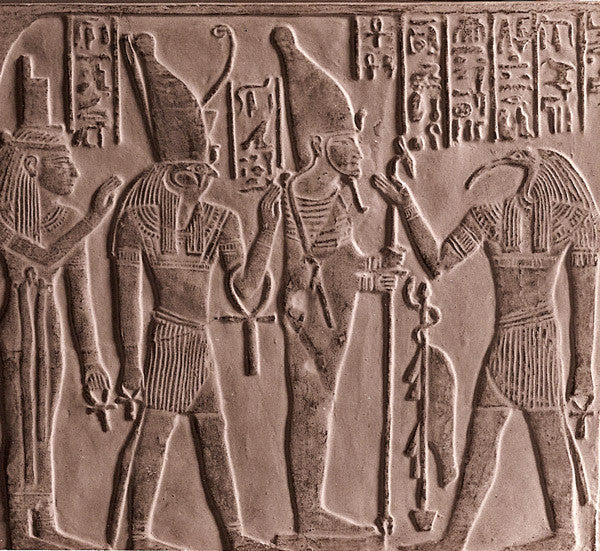The image is an ancient Egyptian hieroglyphic carved into a tan, sandstone-like material. The central focus is on four figures, two of whom appear to be human while the other two have bird-like heads, possibly representing priests or deities. The bird-headed figures, one with a long beak, hold anks and cross-ribbon symbols, which are also worn as bracelets around their elbows. The human figures, adorned in what seems like traditional attire including tall, interesting hats and kilt-like skirts, have raised hands and one of them holds a staff, possibly entwined with a snake. Rows of hieroglyphic symbols and writing tablets are etched above their heads, adding further depth and context to the scene. The entire depiction is rendered in a single terracotta light brown color, emphasizing its ancient and uniform aesthetics.